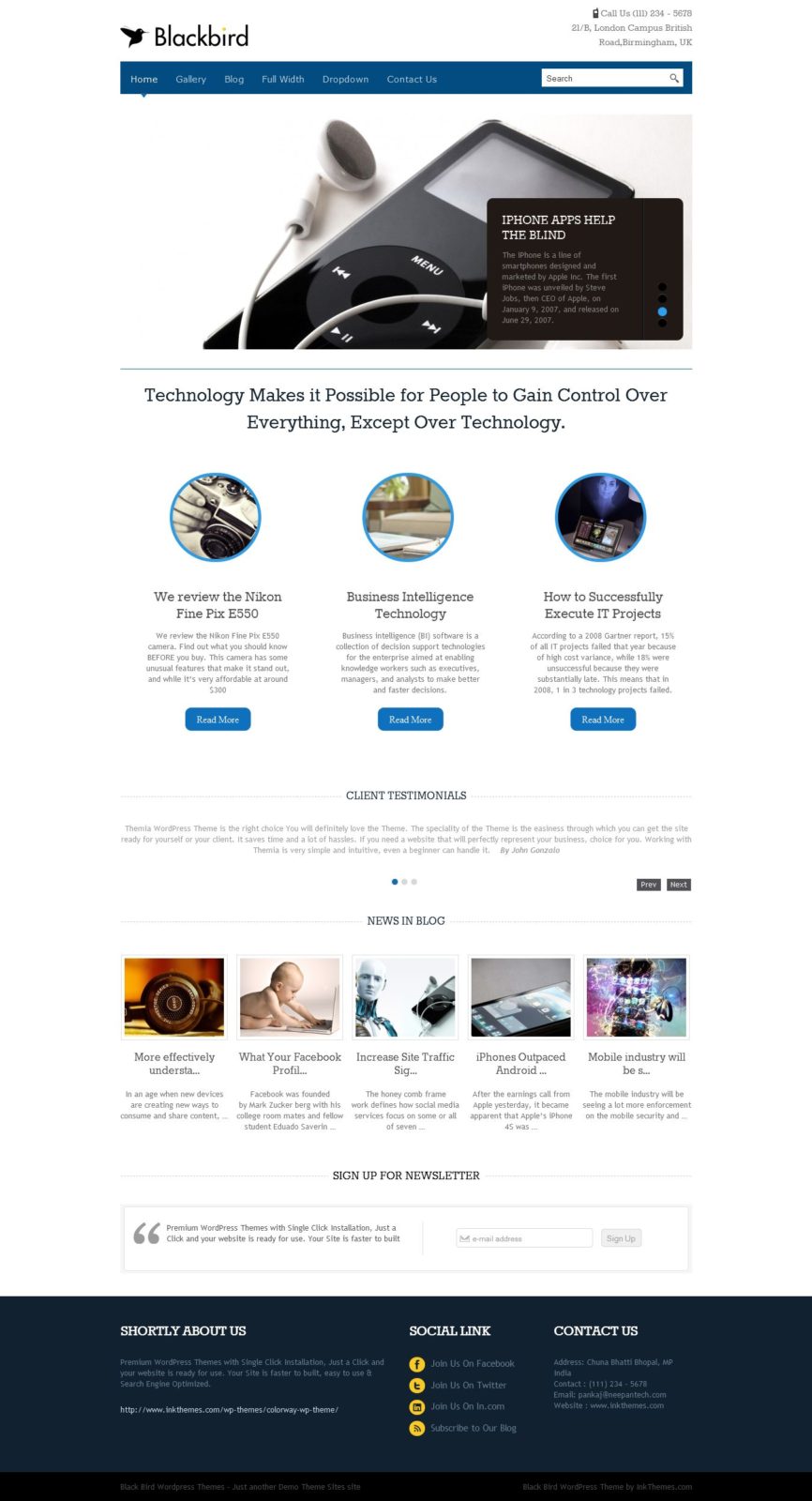The screen capture depicts a website for a company named Blackbird. The primary focus of the site is on iPhone apps that assist visually impaired individuals. The website's main navigation menu at the top includes links labeled "Home," "Gallery," "Blog," "Full Width," "Drop Down," "Contact Us," and "Search."

A prominent quote on the page reads, "Technology makes it possible for people to gain control over everything except over technology."

Below this, three featured articles are listed:
1. A review of the Nikon FinePix ES50.
2. An article on business intelligence technology.
3. A guide on how to successfully execute IT projects.

Each of these articles includes a "Read More" link for further details.

Further down the page, sections for "Client Testimonials" and "News in Blog" appear, displaying additional articles. However, the text in the testimonials section is too small to read clearly.

The website also includes options to sign up for a newsletter, a brief "About Us" section, social media links, and contact information at the bottom of the page.